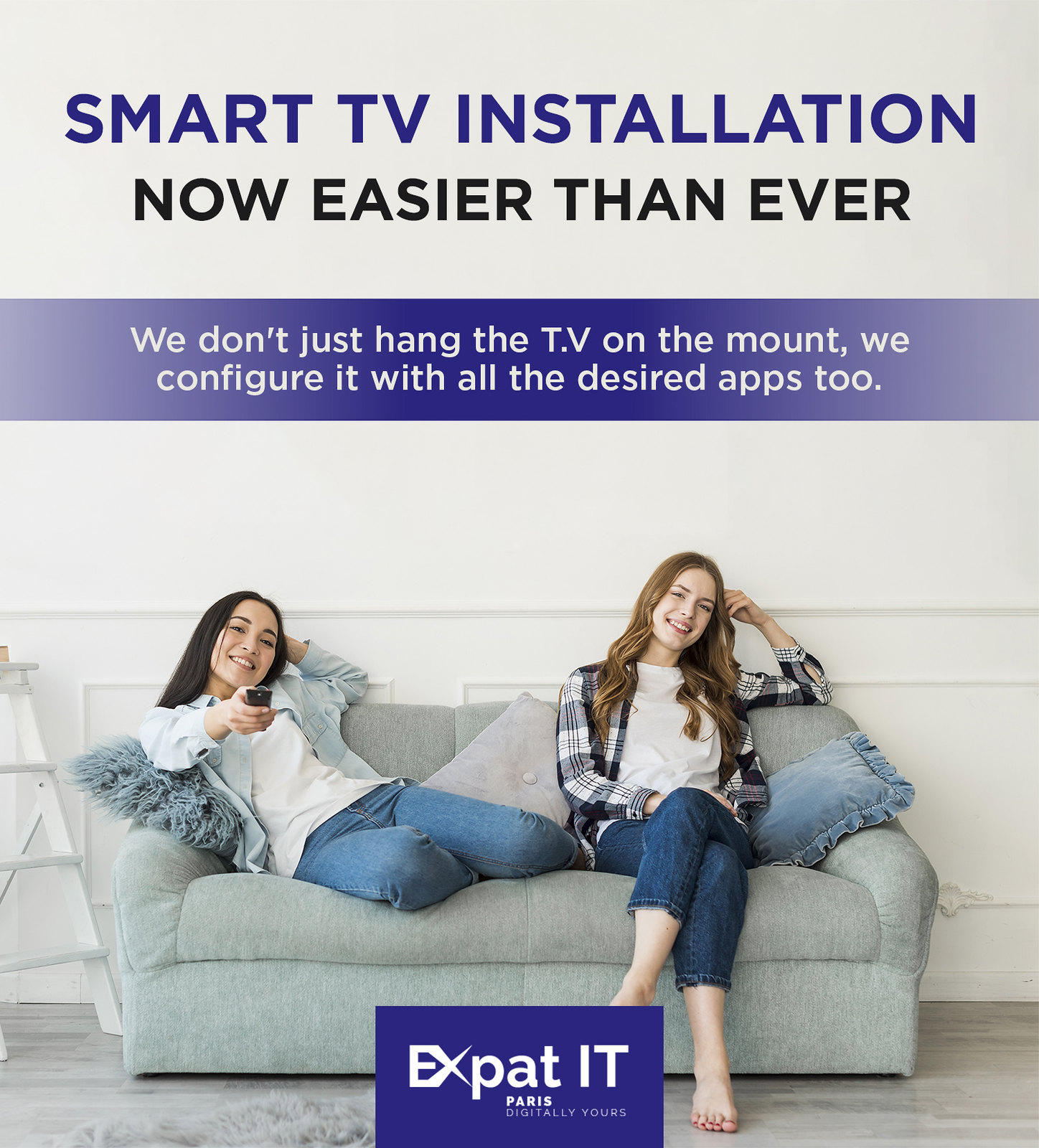In this professionally photographed advertisement, two young women are centrally positioned, sitting comfortably on a light grayish-green couch adorned with numerous pillows. Both are dressed in blue jeans paired with white shirts, with the woman on the left wearing a relaxed denim shirt over her white top and the woman on the right donning an open, darker flannel shirt over hers. Their casual, yet deliberate attire adds to the cozy yet polished ambiance of the setting, which features a clean hardwood floor beneath the couch. The backdrop is a white wall with text in varying shades of blue and black. The upper section of the advertisement prominently displays the slogan, "Smart TV Installation, Now Easier Than Ever," followed by a blue banner with white text that reads, "We don't just hang the TV on the mount; we configure it with all the desired apps too." Towards the bottom of the image, there is a purple or bluish-purple rectangle featuring the logo "Expedit, Paris, Digitally Yours," highlighting the service provider. The overall composition and detailed elements of the scene emphasize the message of effortless and comprehensive smart TV installation.